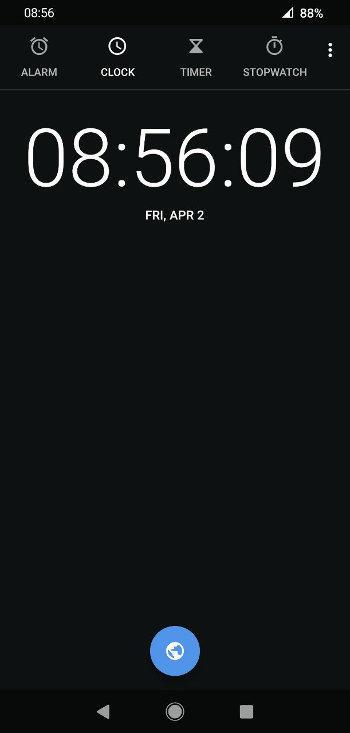The image is a screenshot taken from a cell phone, showcasing the clock application against a solid black background. 

In the upper left corner in white text, the current time is displayed as 08:56. The upper right corner indicates good reception with a signal icon and shows the battery life at 88%.

Below these indicators, the menu options are presented in gray text from left to right:
1. "Alarm" with an icon of a clock above it.
2. "Clock" with an icon of a traditional timepiece above it.
3. "Timer" with a white icon of a timer above it.
4. "Stopwatch" with an icon of a round stopwatch above it.

To the right of these menu options, there are three vertically aligned buttons.

Central to the image, in very large white text, the time is prominently displayed as 08:56:09. Directly below this, in smaller white text, the date is shown: Friday, April 2nd.

The bottom center of the image features a blue home button.